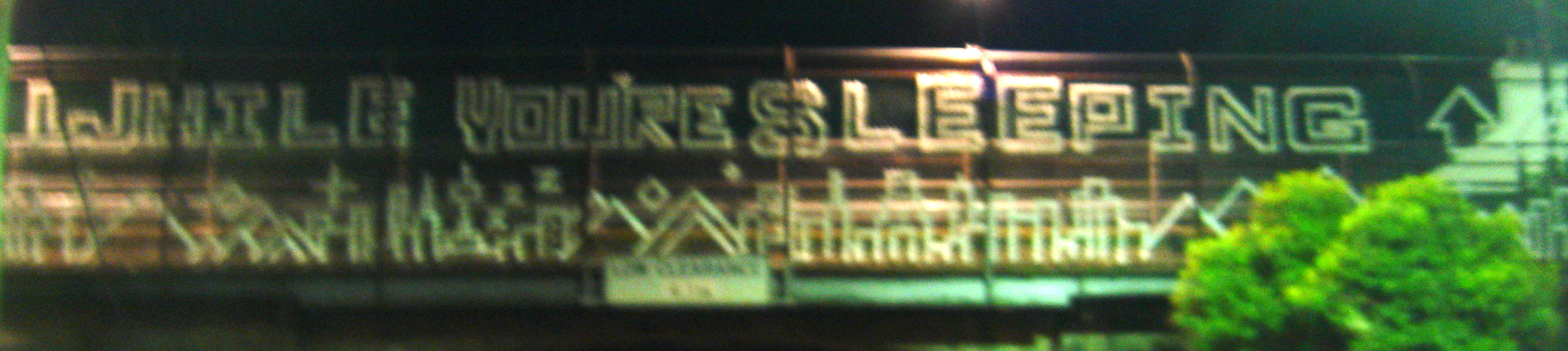The image shows a slightly blurry photograph of a large rectangular sign with a wooden background, running from the left to the right across what may be a fence or the railing of a bridge. The main text on the sign says "while you're sleeping" in block letters with white outlines, above an upward-pointing arrow. Below this text, there is a stylized artwork of an angular town featuring abstract, triangular mountains, and various small buildings also outlined in white. From one of the buildings, three z's are emanating, adding a whimsical sleeping theme. Underneath the town artwork, slightly more out of focus, a small white rectangular sign reads "low clearance." The bottom right of the image shows the tops of some dense foliage, partly obscuring the main sign. The whole image is somewhat blurry, suggesting the camera was moving when the photo was taken, and there are lights aimed at the sign, enhancing its visibility.